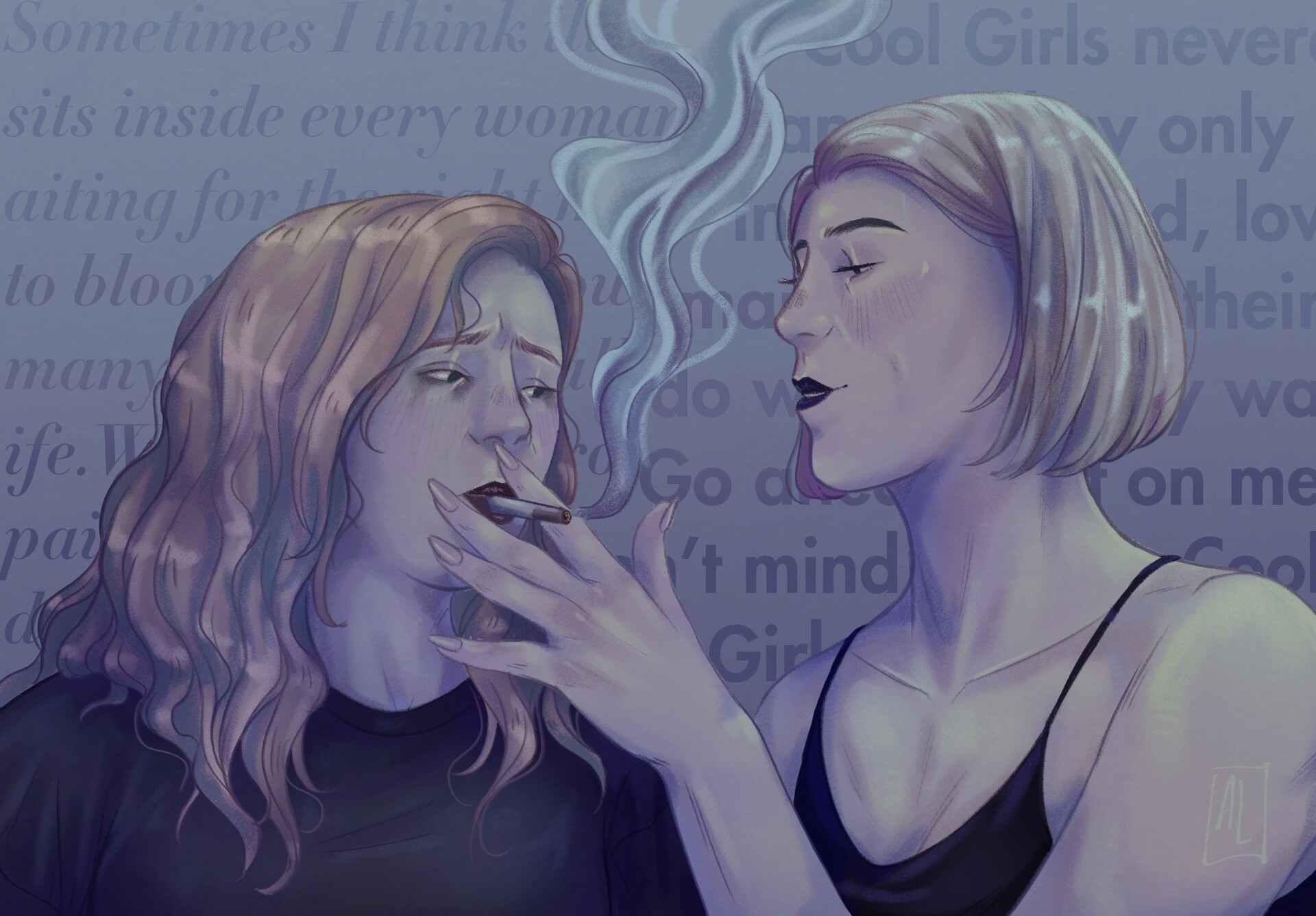This illustration depicts two women in a dark gray, muted-toned setting, with various incomplete quotes as a wallpaper-style background. The woman on the left has shoulder-length, red wavy hair and appears visibly sad, with eyebrows pinched. She is wearing a black shirt. The woman on the right sports a blonde bob hairstyle and wears a black tank top with spaghetti straps, accentuated by dark lipstick. She is holding a lit cigarette to the mouth of the red-haired woman, with smoke billowing between them. The background text includes disconnected phrases such as "sometimes I think it's cool," "girls never sit inside," and "every woman only mind," rendered in two distinct fonts, with some portions written in cursive. The overall scene radiates an atmosphere of melancholy and tension.